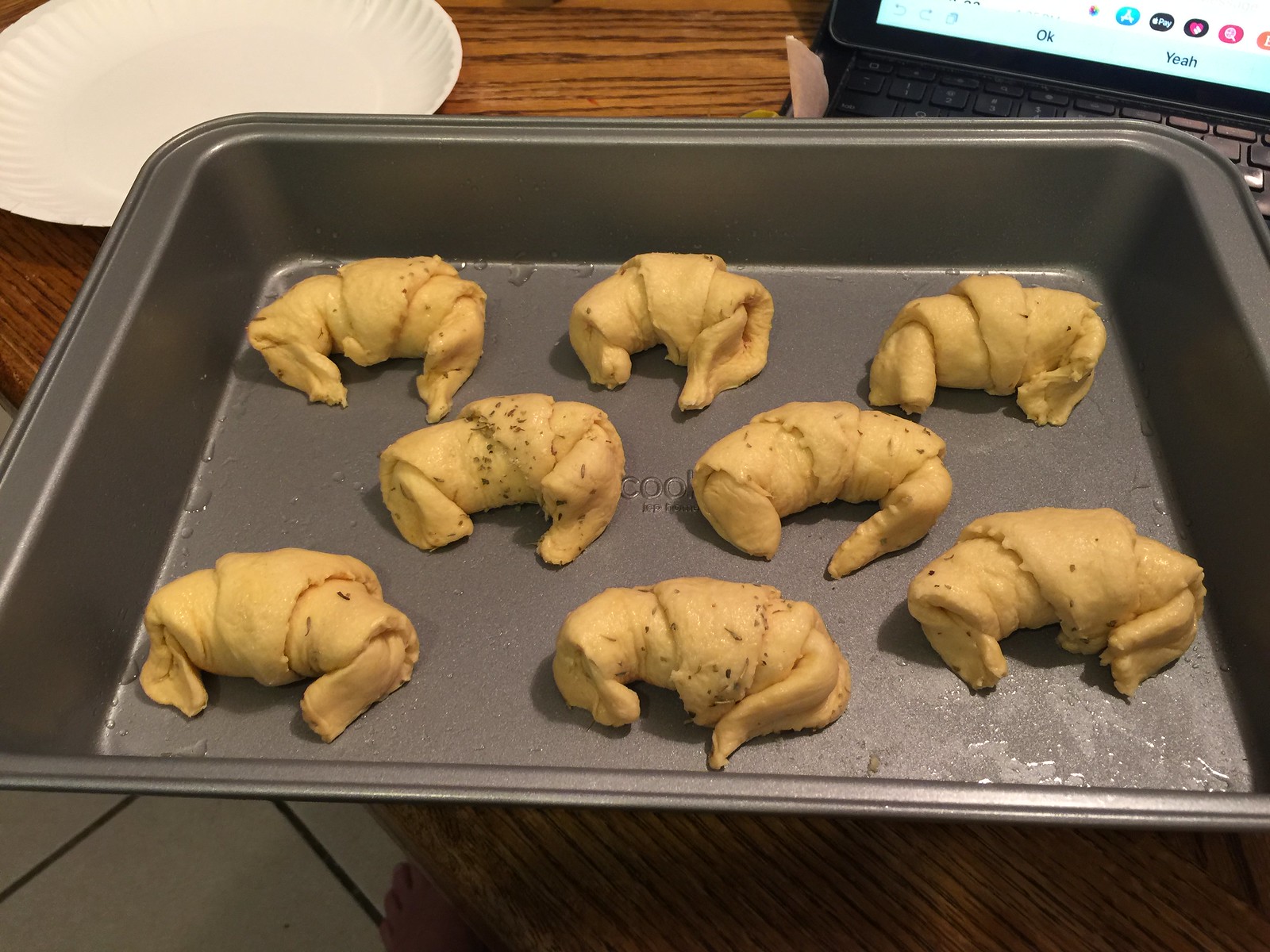This photograph showcases a deep, rectangular, non-stick metal baking pan containing eight uncooked, crescent-shaped dough pieces, arranged for baking. The baking pan, dark grey in color, rests on an oak-colored wooden countertop. Visible moisture inside the pan suggests the crescents have been brushed with oil. A white paper plate is seen in the upper left corner, while the upper right corner features a partial view of a computer screen displaying navigation buttons and icons, including Apple Pay.